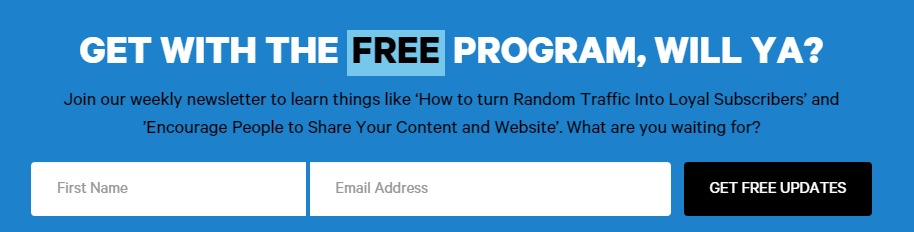A rectangular blue box dominates the center of this minimalistic screenshot. The box prominently features a headline in bold text: "Get with the free program, Lilia." Below the headline, a call-to-action message invites users to join a weekly newsletter. The message promises valuable insights on transforming random traffic into loyal subscribers and motivating people to share content and websites. 

Two input fields are positioned below the message, labeled for "First Name" and "Email Address," inviting users to enter their information. To the right of these fields, a contrasting black button labeled "Get Free Updates" beckons users to complete their subscription. This single-page design is straightforward and focused solely on encouraging newsletter sign-ups.